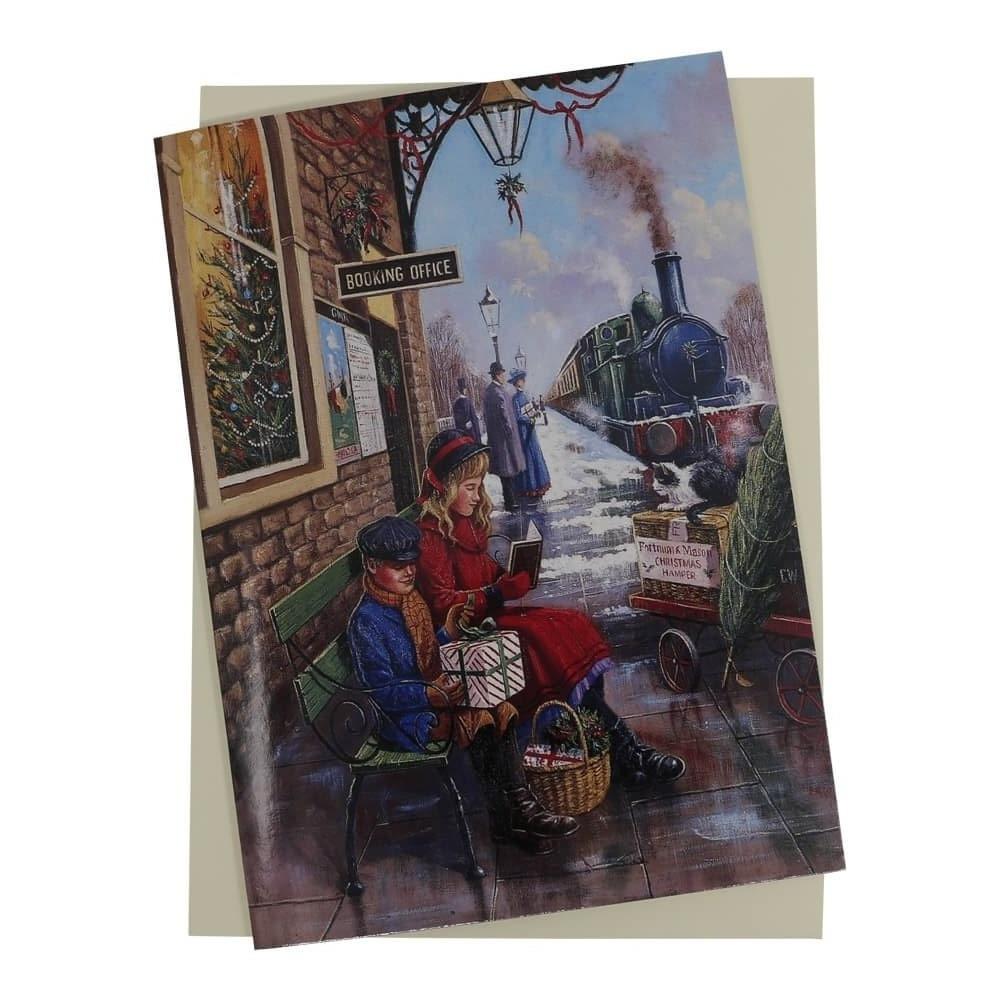In this intricate period drawing, reminiscent of an early 1800s setting that conjures the charm of a Christmas scene, a little girl and a younger boy are seated on a green park bench towards the bottom part of the image, facing to the right. The girl, attired in a long red overcoat and a blue and red hat, is absorbed in reading a black book. Beside her, the boy, clad in a blue jacket and matching hat, holds a present wrapped in green and white striped paper with green ribbons and a bow on his lap. At their feet, a basket filled with gifts and holiday greenery rests on the ground.

In front of the bench, a small red wagon with wagon-like wheels can be seen. On this wagon, a black and white cat sits atop a box alongside a Christmas tree tied to the side. The box bears the words "Christmas something" inscribed on it. Surrounding this scene, the ground glistens as if wet from recent rain, with patches of snow scattered about.

Behind the children, a brown brick building with a window reveals a decorated Christmas tree inside. Above the children, a sign reads "Booking Office." Further in the background, some people gather near an area as a smoking train approaches from the middle to upper right side of the image. The sky is a serene blue with white clouds, completing this picturesque and festive illustration.